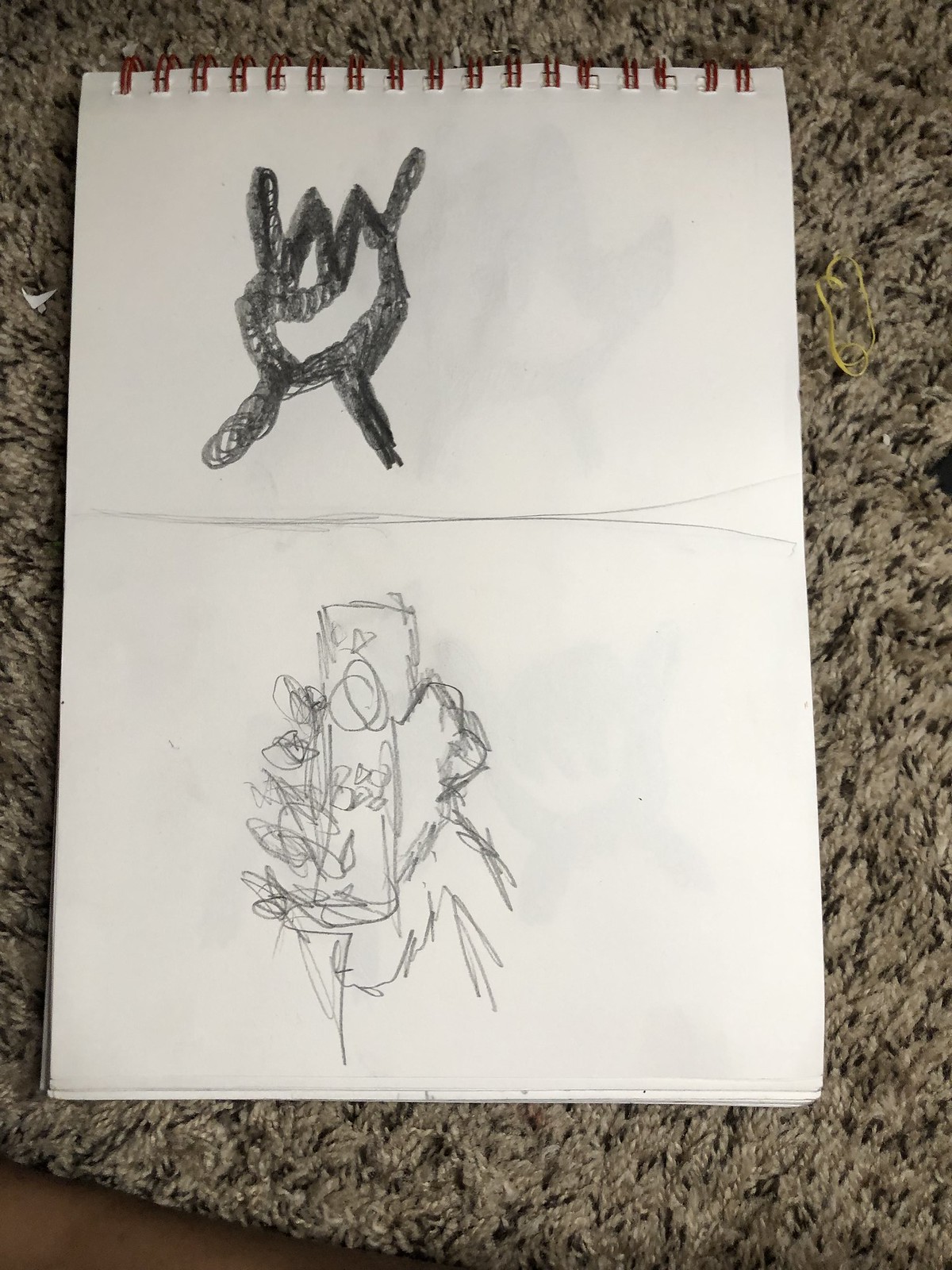This image captures a spiral-bound notebook with brown spirals, lying on a brown, beige, and black shag carpet. A wooden floor peeks from the left corner of the frame. The white pages of the notebook feature two distinct doodles separated by a horizontal pencil line. The top doodle, heavily sketched in dark graphite, appears like a peculiar, spindly-limbed pretzel shape or a hand making an unusual gesture. The bottom drawing, done in lighter pencil strokes, resembles a humanoid figure with a square head, cylindrical body, multiple arms, and two legs. The overall impression is that these scribbles, likely created by a young person, are a mix of abstract and whimsical elements.